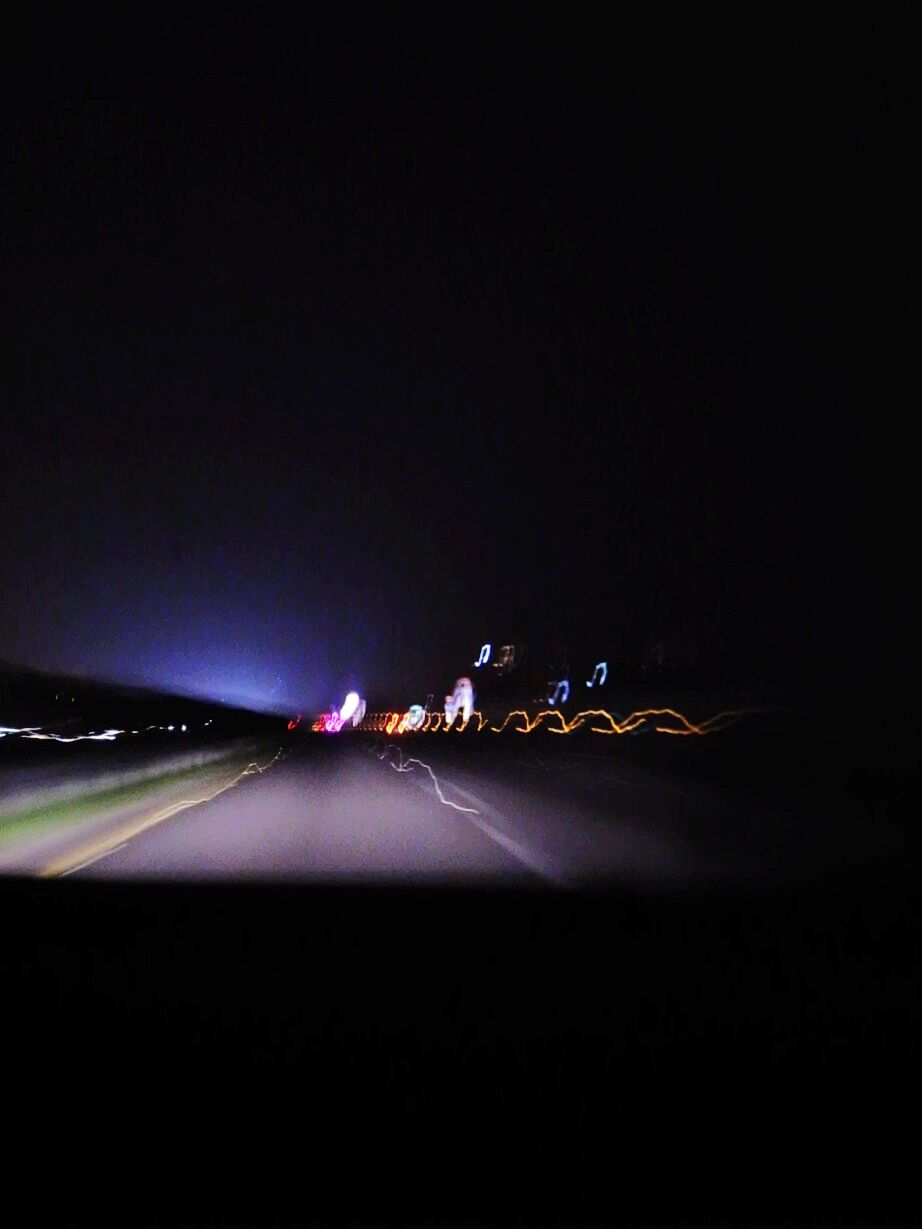In this night-time highway scene, you appear to be seated inside a car, gazing through the front windshield. On the opposite side of the road, a continuous line of solid white lights glows, stretching into the distance. A prominent, large white light illuminates the background. On the right side of the highway, a series of loops of lights are visible, interspersed with various hues. Yellow lights dominate this section, accompanied by small, blue, music note-shaped lights adding a whimsical touch. As the road continues, an array of vibrant lights in shades of yellow, orange, and pink emerge. Towards the end of the road on the right, there seems to be a major attraction, indicated by the clustered, multicolored lights creating a vivid and dynamic display.